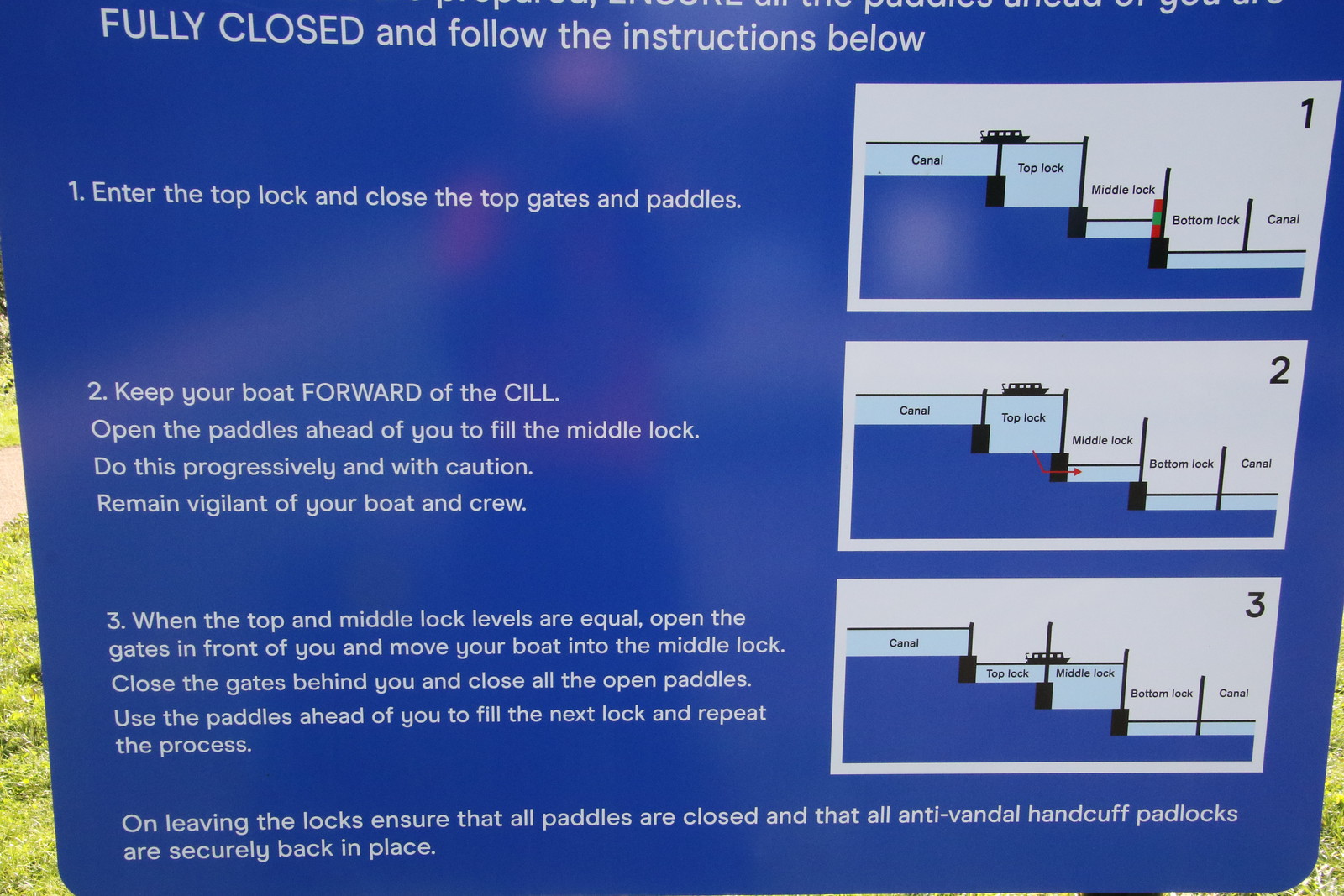The image depicts a blue sign placed outdoors, partially showing grass in the bottom left-hand corner. The sign provides detailed instructions, written in white letters and supported by corresponding images. These three images are labeled 1, 2, and 3 and aligned on the right-hand side. The left-hand side contains step-by-step instructions for navigating a canal lock system.

Step 1 instructs to enter the top lock, then close the top gates and paddles. Step 2 emphasizes keeping your boat forward of the cill, opening the paddles ahead gradually and cautiously to fill the middle lock, and remaining vigilant of your boat and crew. Step 3 explains that when the water levels of the top and middle locks are equal, you should open the gates in front, move your boat into the middle lock, then close the gates behind and all open paddles. Lastly, to create the next lock, you should use the paddles ahead of you and repeat the process. Additional guidance, located at the bottom of the sign, advises ensuring all paddles are closed and anti-vandal handcuff padlocks are secured upon leaving the locks. The images alongside the text visually demonstrate each step, enhancing the clarity of the lock navigation process.